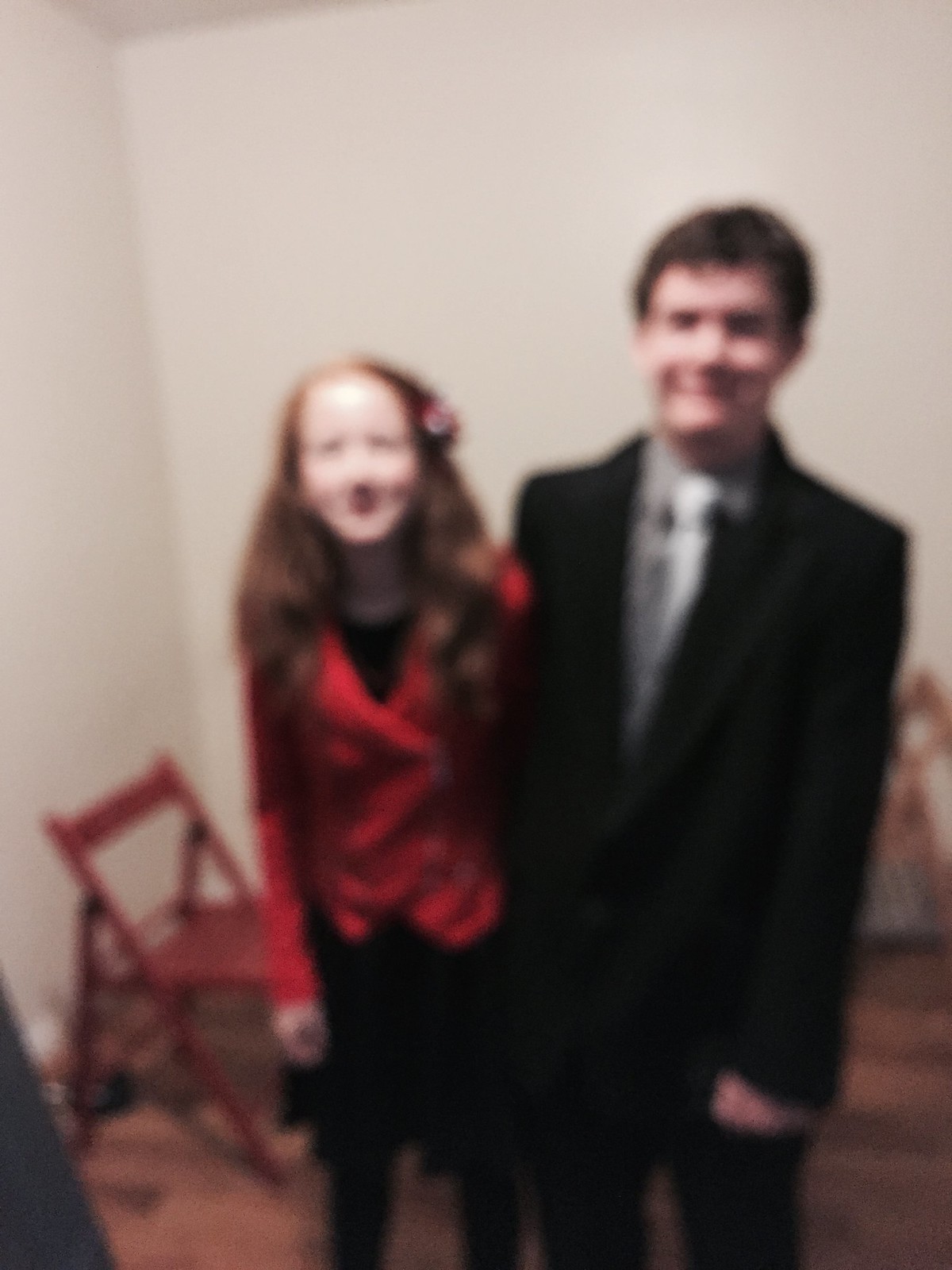This vertically-oriented, slightly rectangular image captures a very blurry interior scene with uneven bright lighting. In the background, there's a white or off-white wall where two walls converge at an upper-left corner, extending downward. The floor, although extremely blurry, seems to showcase a wood grain pattern.

On the lower left side of the frame, a red folding chair is partially visible. The focal point of the image features two individuals standing closely side by side, facing the camera. The person on the right has long, reddish hair that flows over their shoulders and down the chest, complemented by a red long-sleeved top and black pants. Standing to their left, the other individual is dressed in a dark, nearly black suit, with short black hair. This person sports a gray dress shirt with a light gray tie neatly tucked in.

Despite the overall blurriness obscuring fine details, it appears that both individuals are smiling, adding a sense of warmth to the otherwise indistinct scene.